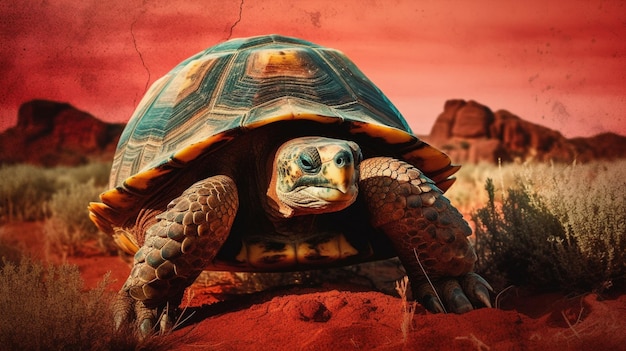In this vivid and detailed image, we see a box turtle in an arid, desert-like environment. The turtle is the focal point, positioned diagonally with its back end towards the left and its front end facing the bottom right. Its shell, a striking green and amber, features a hexagonal pattern, with tan-colored squares bordered by black rings. The turtle's two scaly, brown front legs, equipped with large black nails, are visible as it walks across the red soil. The turtle's face, dappled in yellow and black spots, gazes slightly sideways at the camera, revealing sleepy eyes and one side of its nose.

The background is dominated by a dramatic reddish-orange hue, painting both the sky and the surroundings in a warm, intense tone. Behind the turtle rise imposing rock formation mountains, looking very dry and devoid of grass, punctuated only by sparse, dry shrubs in shades of greenish-brown and yellow. The entire scene, from the red soil to the vivid sky, amplifies the arid, desert-like conditions, creating a visually striking contrast to the intricate patterns and colors of the turtle's shell and scales.